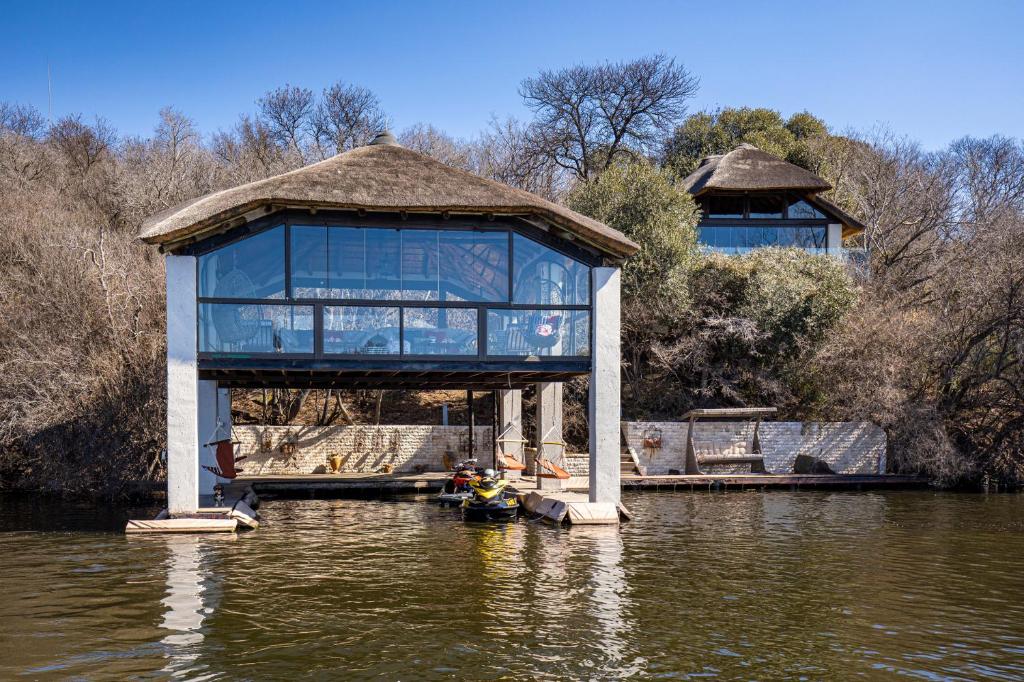In this photograph of a river or lake, we see a dock area where two jet skis, one in yellow and black and the other in red and white, are tied up. The water is a brown, muddied color, suggesting recent rain or churned sediment. The dock is connected to a boathouse-like structure elevated on six pillars, raising it 10-15 feet above the water. The boathouse features large, expansive glass windows all around and is topped with a brown, brush-like or thatched roof. Inside, through the windows, you can glimpse patio furniture. The backdrop is rich with trees, most of which are bare and brown, with a few green ones off to the right. Behind the boathouse, there is a low white brick wall with stairs leading upward, and further in the background, nestled on a slight hill, stands another similar glass-walled building with the same brown thatched roof, partially obscured by trees and bushes.